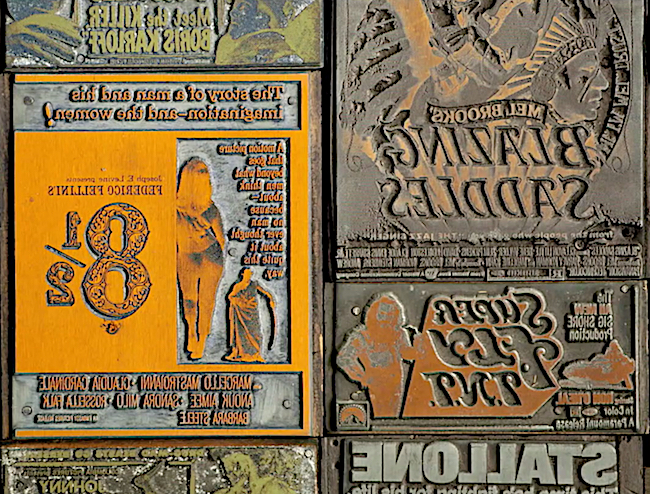This detailed image depicts a close-up view of a collection of aged, etched metal plates designed for stamping or printing purposes, likely on newspaper. The plates, in a vertical rectangular arrangement, feature an array of stamps of varying sizes and shapes, including rectangular and square forms. Notably, these metal etchings, primarily in darkened bronze with hues of yellow, rust, and muted green, display reverse images and text in English, meant to be inverted when stamped to produce the correct orientation.

Among the discernible details, the upper right-hand corner shows an etched image of a chief adorned with feathers on a headband, while on the left side, there is an image of a woman looking away, accompanied by the number 8 1⁄2. The metal surfaces appear somewhat worn, indicating their age and frequent use, and seem to have been mounted on a flat surface, possibly screwed into place. Each plate shares a common theme of backward, raised lettering and imagery, intended to be inked and pressed to convey the correct design on a target medium.